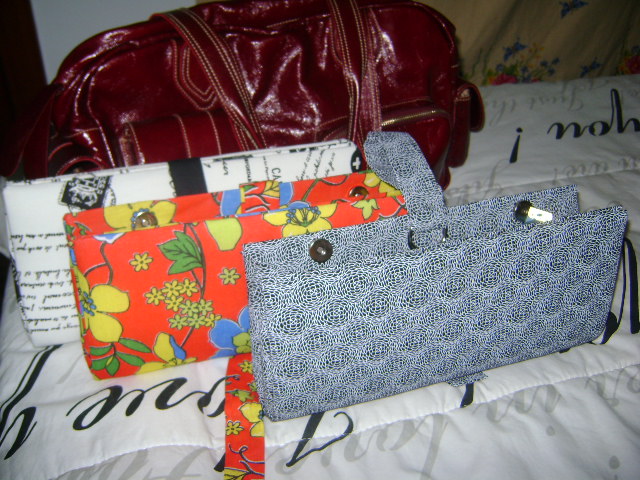This indoor photograph, taken in color, features four distinct handbags artfully arranged on a bedspread. The backdrop of the image is relatively dark, emphasizing the vibrant and varied designs of the handbags. The foremost bag is a smaller wallet-style purse in blue and white, sporting a shell-like design. Behind it is another wallet-style purse with a bright neon orange background adorned with an intricate floral pattern of vines and lemons in yellow and green. Further back sits a black and white wallet-style bag with a newspaper-style print. Dominating the rear is a much larger, rectangular duffel-style bag made from dark red leather, complete with white accent stitching and a long handle that swoops elegantly behind the smaller purses. The handbags, seemingly custom-made, are purposefully laid out in a diagonal arrangement from right to left, suggesting that this image may be intended for selling the items online.